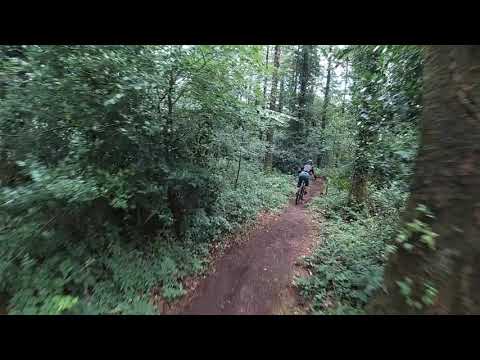Inside a lush forest, a solitary dirt path winds through towering green trees, their thin trunks stretching skyward and creating a canopy that partially obscures the blue and white sky above. The path, brown and slightly muddy, is flanked by short plants, grass, and scattered small shrubs, including clover-like foliage. A cyclist, dressed in casual gear with a blue helmet, grey top, blue pants, and white shorts, rides a dark-colored mountain bike, moving away from the camera and curving slightly to the right. The forest floor is dotted with old, brown leaves, and the overall scene is bathed in the soft light of early morning or mid-afternoon, adding a gentle blur to the vibrant greenery. The serene setting is visually captured, possibly through a bodycam or GoPro, offering an immersive glimpse into this tranquil biking adventure.